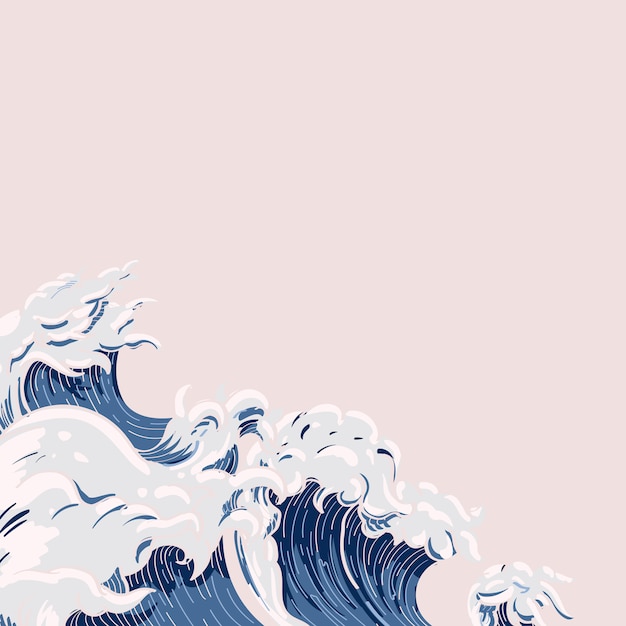The image depicts a simple yet evocative drawing of ocean waves set against a plain, subtly light pink background. The waves are largest on the lower left side of the image, with frothy, white tips that gradually diminish in size as they move towards the right, ending just before the lower right-hand corner. The waves are primarily dark blue but feature streaks of lighter blue and faint pink hues from the background. The striking white water at the crest of the waves forms a distinctive splash effect, giving the scene a sense of dynamic movement despite its simplicity. The uniform pink background lacks any additional elements such as the sky or beach, further emphasizing the waves' motion and formation.